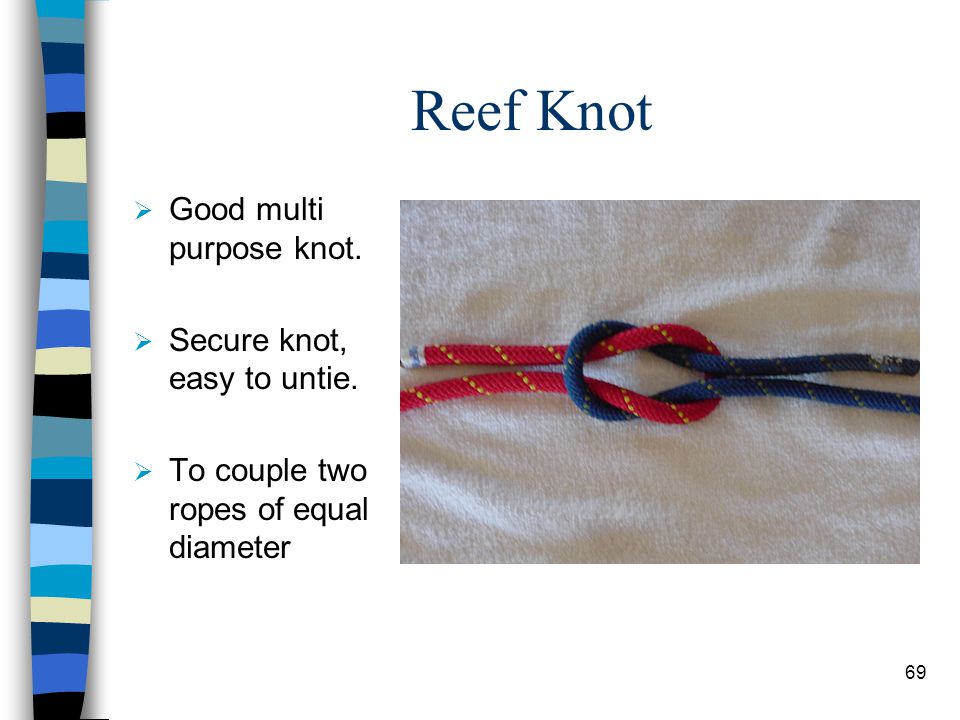The image is a photograph portraying a Reef Knot, presented in the style of a PowerPoint slide. The background appears white, and on the left side, there is a vertically oriented, segmented band with various horizontal color sections including shades of blue, dark blue, gray, tan, and black. The headline at the top, in large blue font, reads "Reef Knot," indicating the type of knot depicted. The knot itself is positioned centrally but slightly to the right of the image, tied using one red rope and one blue rope, both seemingly laid on fabric. There is descriptive text on the left and the top which details the knot’s characteristics: "Good Multipurpose Knot," "Secure Knot," "Easy to Untie," and "To Couple Two Ropes of Equal Diameter." Additionally, the number 69 is marked in the bottom right corner of the image.